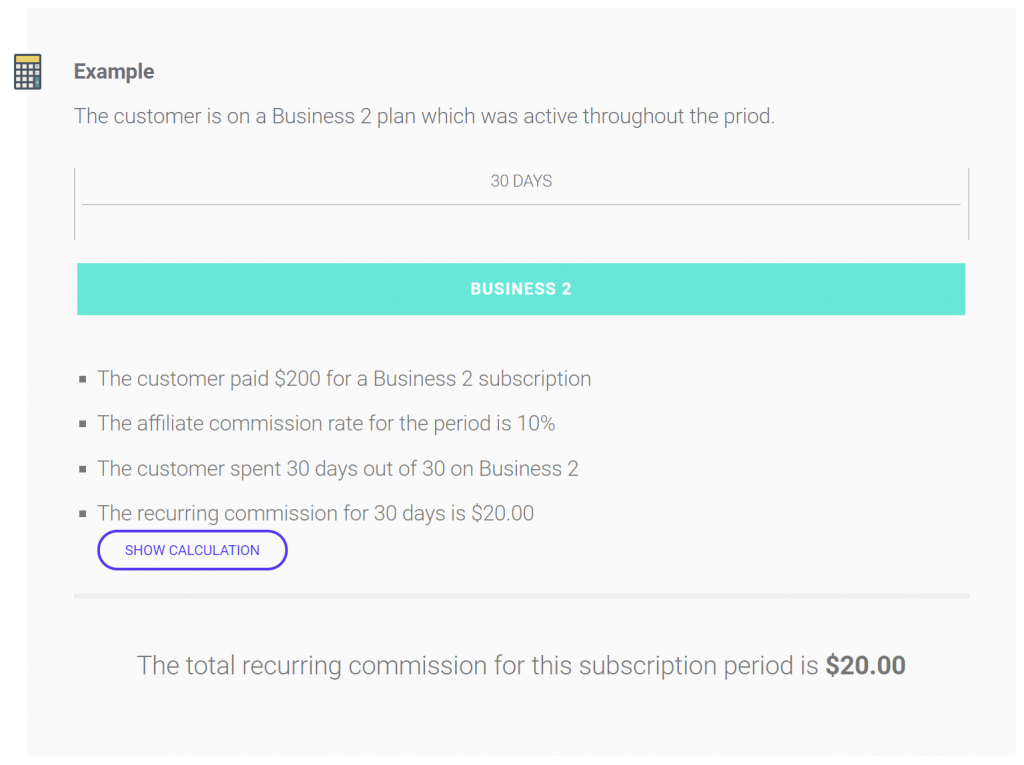This image depicts a sample web page for a business plan. In the top left corner, the word "Example" is prominently displayed. To the right of this text, there is a noticeable space followed by an icon resembling a calculator. Below the icon, a sample block is visible with additional empty space around it.

Further down, in a grayish font, it states that the customer is on a "Business Plan" which is active for the period. Below this text is the phrase "30 Days," which is centrally aligned. 

A thin, gray separator bar spans from left to right below the "30 Days" text, followed by a light green bar of the same width. In the center of this green bar, the words "BUSINESS PLAN" are inscribed in white, all-caps font.

Situated under this green bar are four bullet points that are left-aligned. Beneath these points is a button labeled "Show Calculation." At the bottom of the page, it mentions the total recurring commission for the subscription period, which amounts to $20.